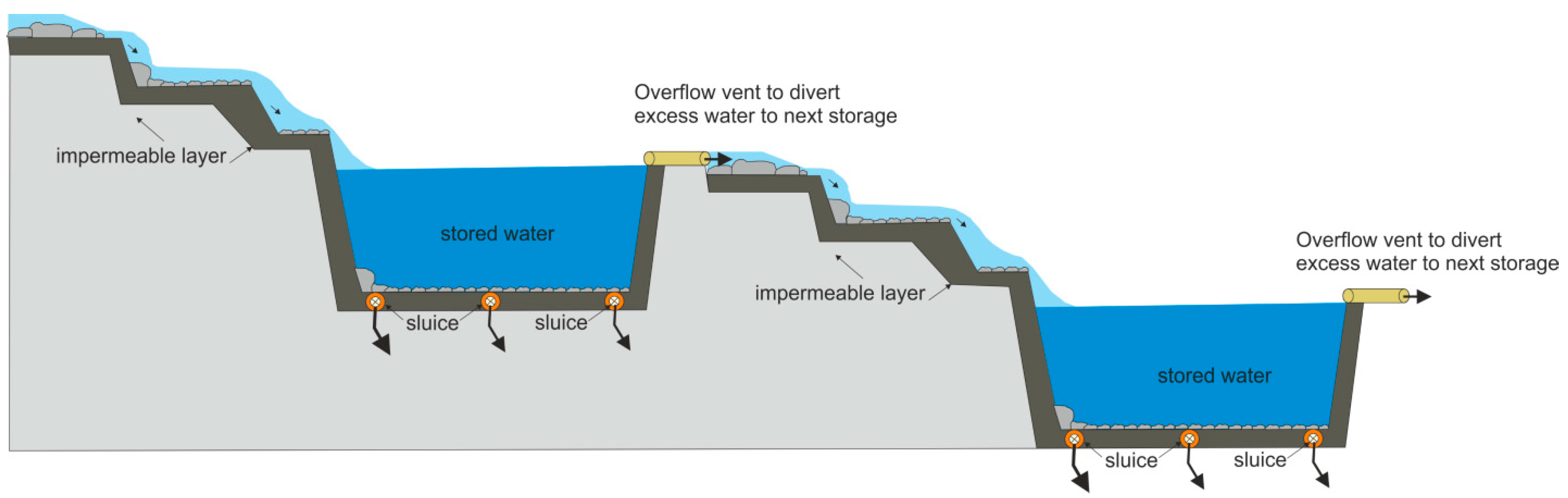This technical illustration demonstrates the process of storing water runoff over a sloping terrain. The diagram begins on the left side, depicting water flowing downhill into multiple storage basins. At the top of the image, there is a label pointing to the flowing water that reads "impermeable layer." The illustration shows water trickling down into a first stored water tank, which is visibly blue and marked as "stored water." Below the stored water tank, text indicates an "overflow vent to divert excess water to next storage," with arrows directing the flow of water downward to the subsequent storage basin. This pattern repeats, with each segment displaying an impermeable layer beneath the water, additional stored water tanks, and overflow vents guiding excess water down the slope into the next storage area. The illustration methodically details the movement and management of water runoff through a series of reservoirs to ensure efficient storage.